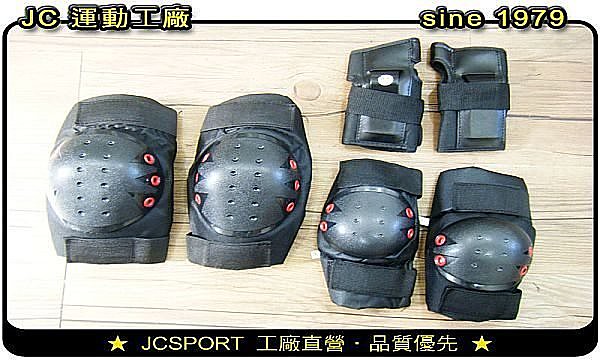This image showcases a collection of black sporting gear, including knee pads and wrist pads, arranged on a light wood floor. The knee pads feature circular padding with small, detailed rivets and red holes. The wrist pads have black straps and similar red accents. The floor varies in description, being referred to as a rough light wood or pine. The upper right corner of the image includes the text "sign, S-I-N-E, 1979," while the top left features the initials "JC" followed by characters in a foreign language. The bottom of the image contains a black banner with two yellow stars and the text "JC Sport" accompanied by more foreign characters. The overall image is bordered in black, reflecting light slightly off the objects.